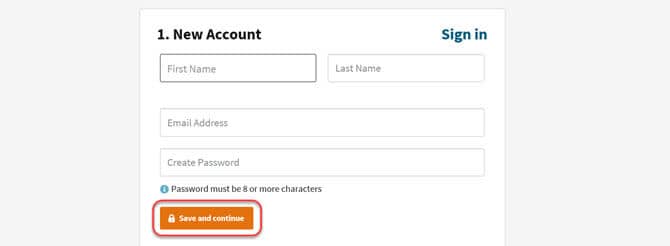This image is a cropped screenshot from a webpage, displaying a section of an account creation form. The overall shape of the image is a rectangle, with a very light gray background. In the center of this rectangle is a white square, presumably the main content area of the form. 

At the very top left corner of the white square, there is the text "1. New Account" in black font. On the opposite side, at the top right corner, the text "Sign In" is displayed in blue font.

Below this header, the form contains two horizontally aligned rectangles outlined in gray. The rectangle on the left is labeled "First Name," and the one on the right is labeled "Last Name." Beneath these rectangles, a larger rectangle outlined in gray is labeled "Email Address." Directly below this, there is another similar rectangle that is labeled "Create Password." Under the password field, there is a note in plain text stating, "Password must be 8 or more characters."

Towards the bottom left of the form, there is an orange rectangular button with white font that reads "Save and Continue." This button is highlighted by a red outline drawn specifically around it, drawing attention to its significance on the form.